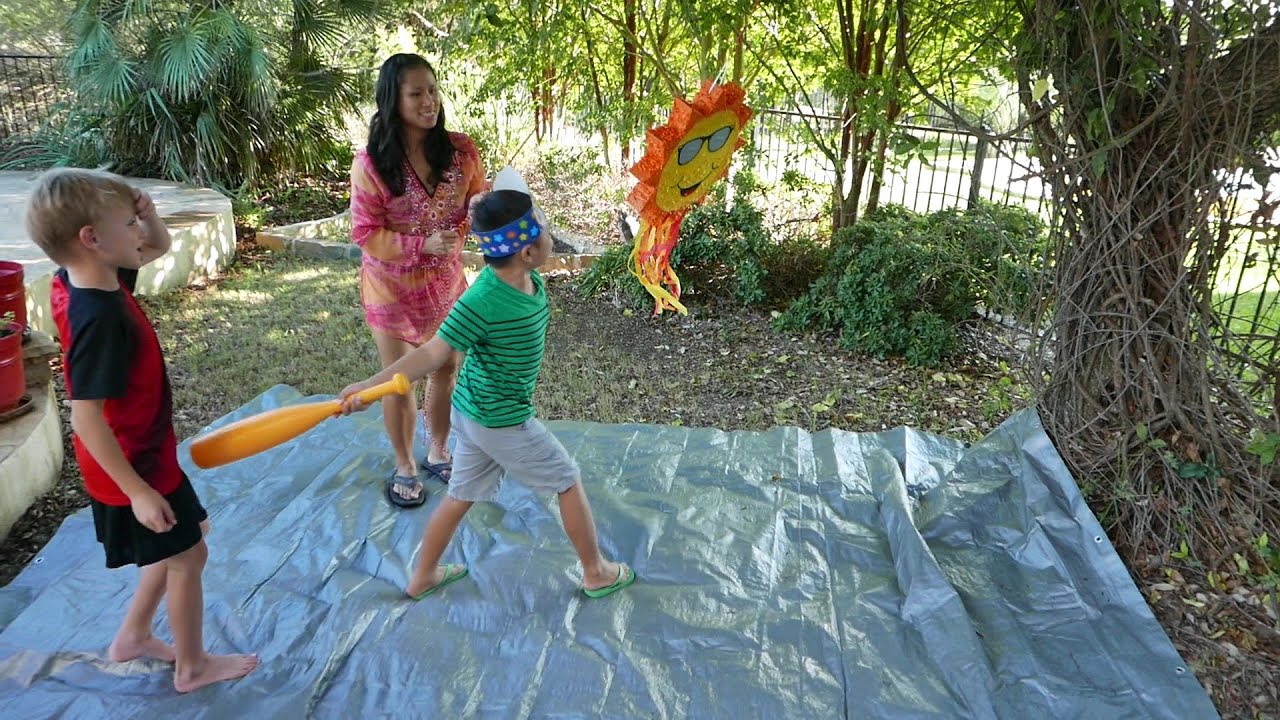This photograph captures a lively outdoor party in a backyard setting, surrounded by lush greenery, including towering trees and vibrant bushes. A metal fence, approximately waist-high, runs along the background. In the foreground, a large blue plastic tarp is spread across the ground beneath a prominent tree with thick vines at its base. Hanging from a branch of this tree is a festive piñata shaped like a smiling sun, adorned with sunglasses, featuring orange rays and a yellow center, with yellow and red streamers trailing from its base.

Centered under the piñata, a young boy stands poised to take a swing. He is dressed in a green and black-striped shirt and khaki shorts and wears a blindfold. Holding a yellow bat in his right hand, he readies himself to hit the piñata. Standing nearby, a woman with long dark hair, clad in a vibrant pink-orange dress with black sandals, watches with a joyful smile, likely encouraging her son. Off to the left, at the edge of the tarp, another young boy patiently waits his turn. He has blonde hair and is wearing a red and black shirt with black shorts. The backyard scene is bustling with anticipation and excitement.